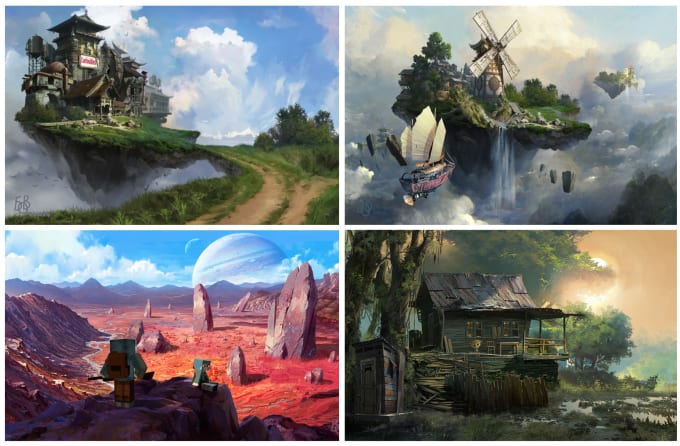A color painting collage arranged in a two-by-two grid, each piece equally sized, depicts varied and imaginative landscapes. The top left painting showcases a futuristic, fantasy scene with a blue sky dotted with white clouds, green grass, and an elevated house perched on a cliff on a floating island, with a dirt roadway winding upwards. Adjacent to it on the top right, a similar scene features a windmill on another floating island, joined by vivid green lawns and cascading waterfalls, with a ship bearing sails approaching the island. The bottom left illustrates an extraterrestrial setting reminiscent of Mars, characterized by red soil, rock formations, and a large, distant planet in the blue, cloud-streaked sky. Several small robot-like figures dot the landscape, highlighting the scene's surreal, habitable quality. The bottom right painting captures a more realistic swamp environment, focusing on a rustic wooden cabin with metal sheet roofing, surrounded by green trees and bathed in the soft glow of a setting sun, casting an orange hue across the sky.